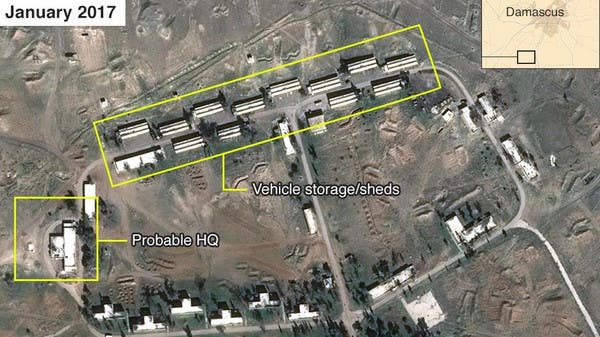This aerial photograph, taken in January 2017 and labeled "Damascus, Syria" on the right side, captures a detailed view of a compound. A prominent yellow rectangle outlines a line of hangars in the center of the image, labeled in yellow text as “Vehicle Storage/Sheds.” To the left of these hangars, another yellow square highlights a building labeled "Probable HQ" in white text. Surrounding these highlighted buildings are various unlabeled structures, visible on the right and lower-left sections. The area also features roads, craters, and a line of trees in the bottom left, indicating signs of prior activity or bombardment. This detailed imagery appears to have been taken by a high-altitude reconnaissance platform, potentially a spy plane, satellite, or drone, and seems designed to keep track of these locations for strategic purposes.